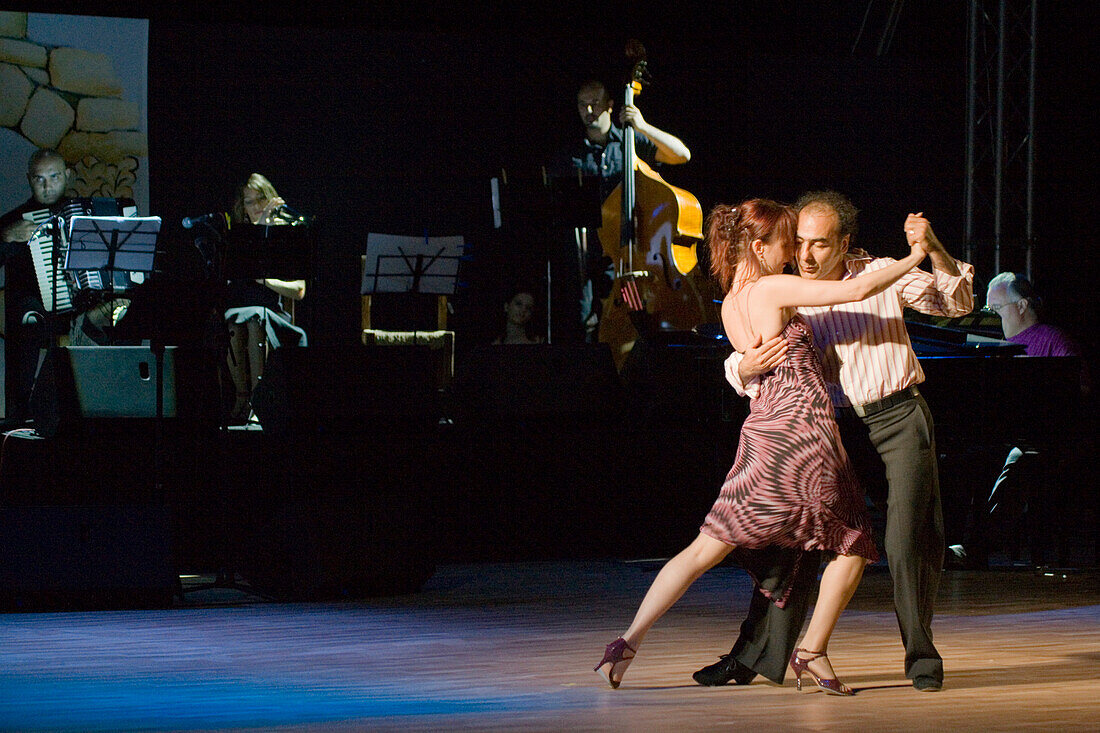This photograph captures an intimate moment between two dancers, spotlighted on a dimly lit wooden dance floor inside a club. The scene appears to feature professional tango dancers performing against a mostly black background bathed in subtle blue lighting. To the left, an orchestra adds live music to the ambiance; it includes an accordion player reading from a music stand, a partially obscured female musician, and a prominently visible upright bassist.

In the foreground, an older, partially bald man with black hair is dressed in a striped long shirt and gray pants, dancing closely with a middle-aged woman who has her reddish-brown hair pulled back in a ponytail. She wears a sleeveless, strapless dress with geometric patterns in shades of red, brown, and white, paired with high-heeled brown shoes. Her attire and posture suggest elegance and poise as they glide through their dance steps. To the right, adding to the rich musical backdrop, a pianist can be seen, while above the main performers, a musician plays a large bass. The detailed attention to their attire and the instruments surrounding them enriches the photograph with a dynamic and lively atmosphere.